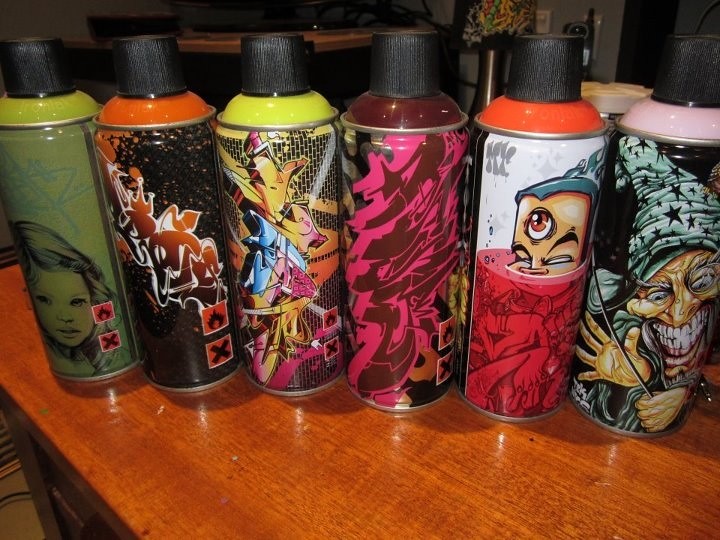This indoor photo captures a close-up view of six vividly colorful spray paint cans arranged on a highly reflective, glossy wooden table with a red sheen. Behind them, hinting at the setting, is another table holding a bouquet of flowers and a pink object. Each can has a distinct design and a black lid. From left to right: the first can is green with an illustration of a little girl; the second features an orange and black flame pattern; the third is yellow with additional magenta and blue designs; the fourth is black with a pink design; the fifth is burgundy with a white top and an orange stripe, displaying a caricature of a man's head submerged in red liquid with a prominent third eye; the final can is black with a pink top, depicting an old witch with white hair, a turquoise hat adorned with stars, and bared teeth. The detailed designs and vibrant colors of the cans are strikingly set against the glossy, reflective surface of the table.